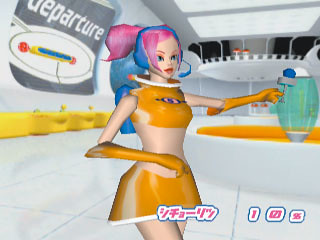The image depicts a brightly colored, computer-generated scene with a young woman prominently featured in the foreground. She is dressed in a vivid, futuristic ensemble reminiscent of the style seen in "The Jetsons." Her outfit includes an orange skirt, an orange top that reveals her midriff, and long orange gloves that extend up to her elbows. Her pink hair is styled in a ponytail, and she wears a blue headset, adding to her modern and tech-savvy appearance.

In the background, a gray sign with the word "Departure" written in white letters is visible, suggesting a transportation hub or futuristic terminal. The sign also features an oval element, though its contents are indiscernible. Beyond the sign, a raised walkway enclosed in glass can be seen, lending a further sense of a high-tech, futuristic setting.

Additionally, there are some red and white characters bordered by blue at the bottom of the image; however, the characters appear to be in a foreign language and are not legible. The overall scene exudes a vibrant and advanced atmosphere, blending elements of retro-futurism with modern digital art.